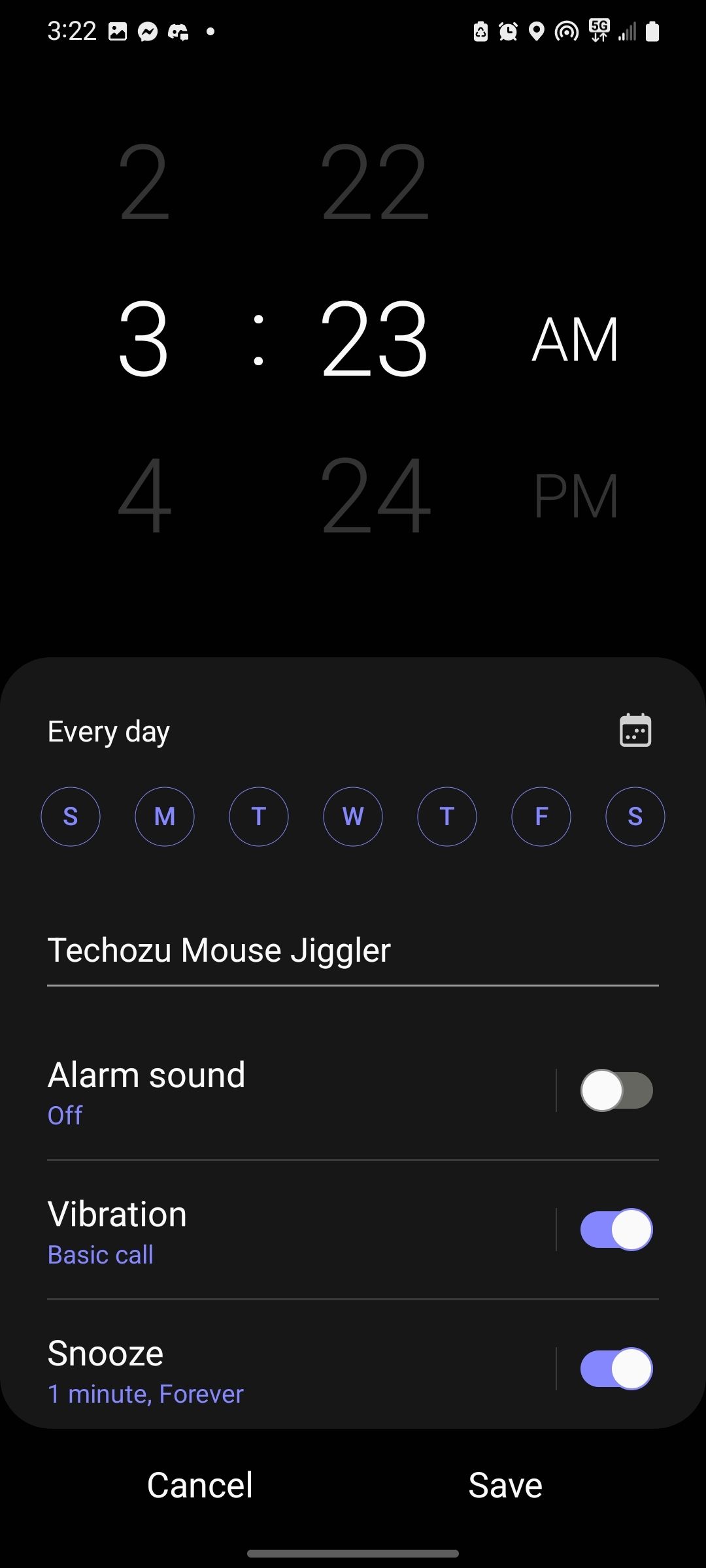The image depicts a smartphone screen in portrait orientation with a predominantly black background. On the top-left corner, the time "3:22" is displayed, accompanied by a small picture icon and the Discord app icon. In the top-right corner, there are several status icons including an alarm clock, a marker, a hotspot icon, the "5G" network indicator, a reception icon, and a battery level icon.

Below this status bar, in large white numbers, the time "3:23 a.m." is prominently shown, suggesting an active alarm set for this time. Above this, the gray text "2:22" is displayed, while below it, another gray text reads "4:24 p.m."

A darker gray box is positioned beneath these time indicators, labeled "Every day." Within this box, the initials "SMTWTFS" are each enclosed in circles, representing the days of the week.

Further down, the screen shows options related to the alarm: "Tetcho Mouse Jiggler Tetcho Zoo" appears, followed by "Alarm sound," which is set to "Off," with a corresponding gray toggle button. "Vibration" is set to "Basic call," with its toggle button being blue. The "Snooze" function is set to "One minute forever," and its toggle button is blue as well.

At the very bottom of the screen, there are two buttons: "Cancel" on the left and "Save" on the right.